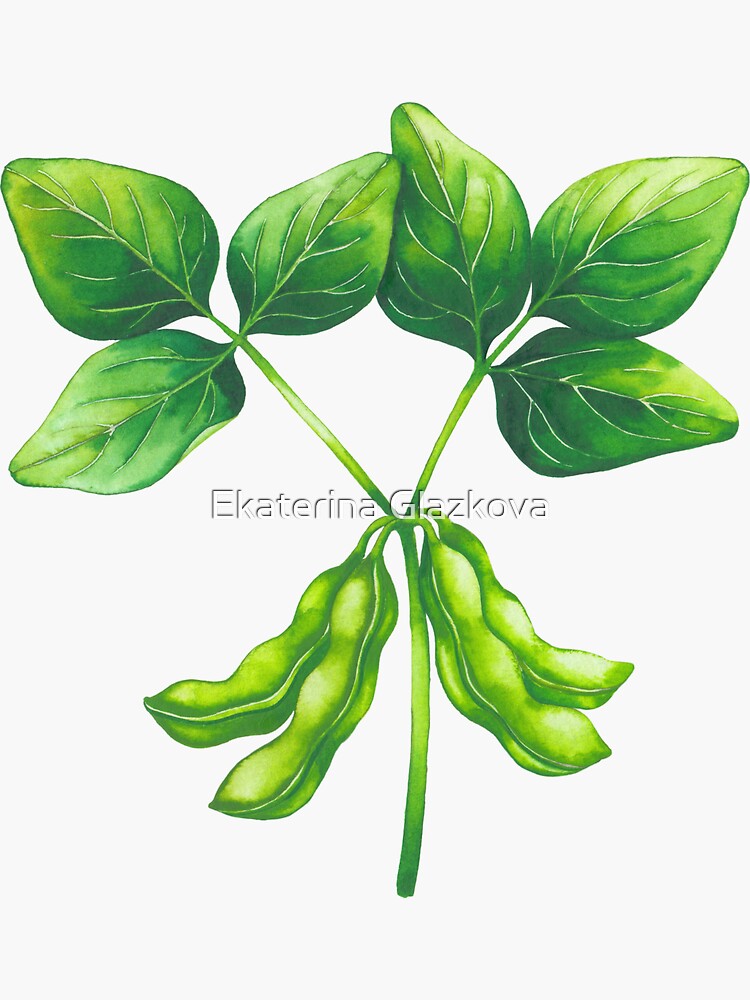This generated image showcases a vertically aligned stem that initially appears green, transitions to yellow, and then reverts back to green. At the center of the vine, two peapod-shaped structures branch out symmetrically on each side, blending hues of green and yellow. The name "EKATERINA GLAZKOVA" is prominently featured in the center. The stem further divides at the top into two branches—one extending to the left and the other to the right. These branches exhibit a sequence of green, yellow, white, and green colors. Each branch supports three leaves, displaying varying shades of darker and lighter green. The entire design is set against a pristine white background, accentuating the vibrant colors.